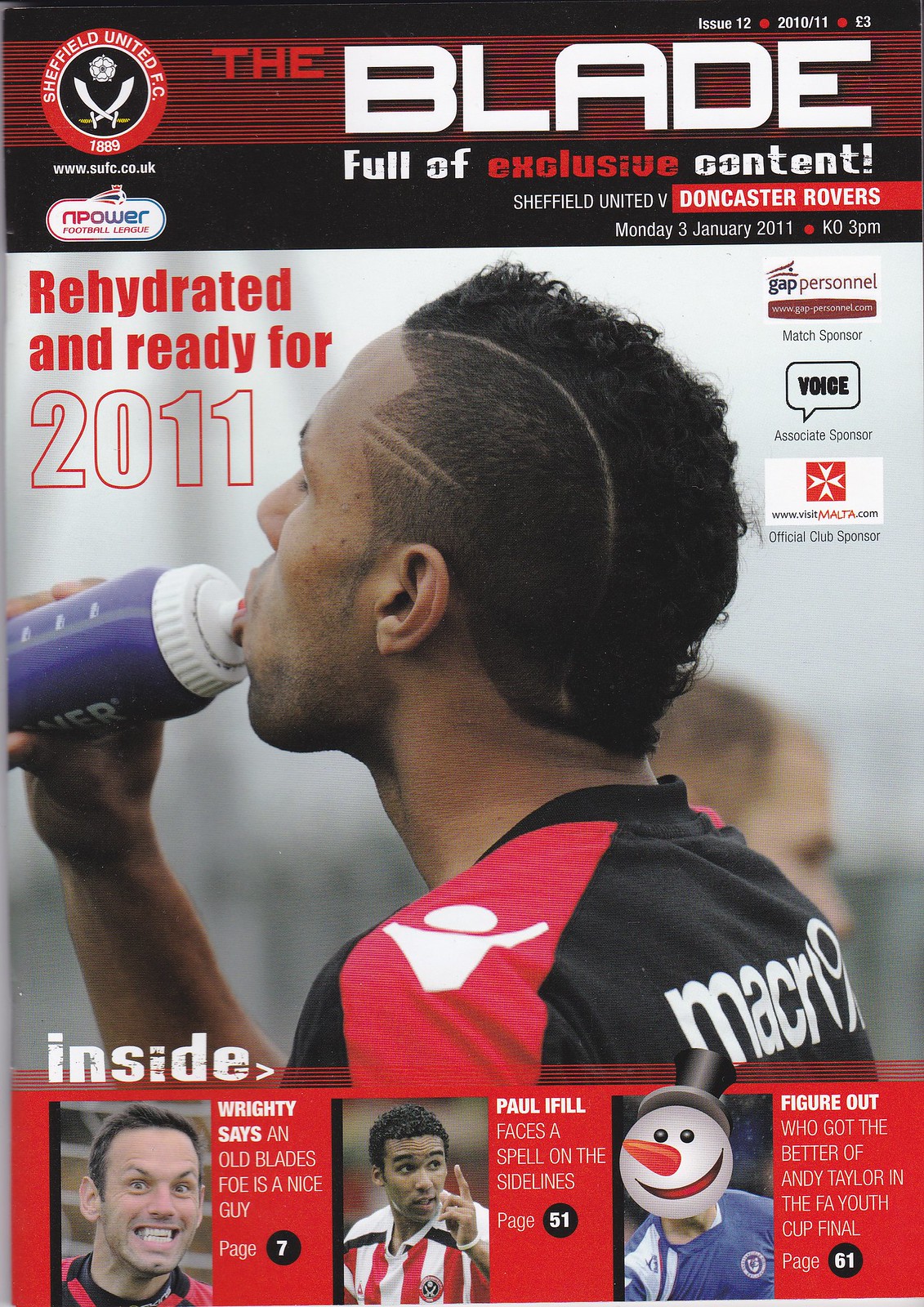The cover of the magazine titled "The Blade, Issue 12, 2010-2011" features exclusive content for Sheffield United FC. It includes details of the match against Doncaster Rovers on Monday, January 3, 2011, with kick-off at 3 p.m. The magazine, priced at £3, shows an athlete on the cover, drinking from a water bottle and facing to the left, wearing a black, red, and white shirt with visible sponsors on the right. The bottom section displays three smaller images: the first is of a man smiling, the second shows another man pointing to the side, and the third depicts a person with their face obscured by a snowman head. The captions reveal additional content, such as "Inside, Righty says an old Blades foe is a nice guy, page 7," "Paul Ifill faces a spell on the sidelines, page 51," and "Figure out who got the better of Andy Taylor in the FA Cup final, page 61." The issue also hints at Sheffield United being "rehydrated and ready for 2011."